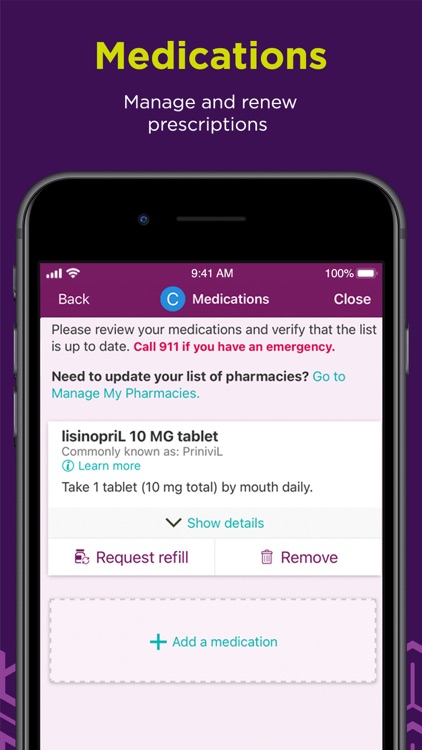**Detailed Caption:**

The image features a smartphone with a purple background, overlaid with detailed informational text regarding medication management. At the top of the image, the word "Medications" appears in yellow text, followed by "Manage and renew prescriptions" in white text.

On the phone's display, a purple bar is positioned at the top. On the left side of this bar, the word "Back" is displayed, and in the center, "Medications" is written next to a blue circle containing a white letter "C." To the right, the word "Close" appears in white text.

The main screen of the phone is white, displaying the message: "Please review your medications and verify the list is up to date." This is written in black text. Below, in pink text, it reads, "Call 911 if you have an emergency." Further down, in black text, it asks, "Need to update your list of pharmacies?" This is followed by a blue text link stating, "Go to manage my pharmacies."

In the content area, there is a box containing a prescription detail, which reads: "Lisinopril 10 mg tablet, commonly known as Prinivil." Next to this, there is a blue circle with an "i" inside, and the text "Learn more" in blue. The prescription instruction below states: "Take one tablet (10 mg total) by mouth daily," in black text. A blue downward arrow indicates "Show details."

Further options include "Request refill" and "Remove," both in purple text. At the bottom, there is a checkered button with the text "Add a medication" in greenish-blue text.